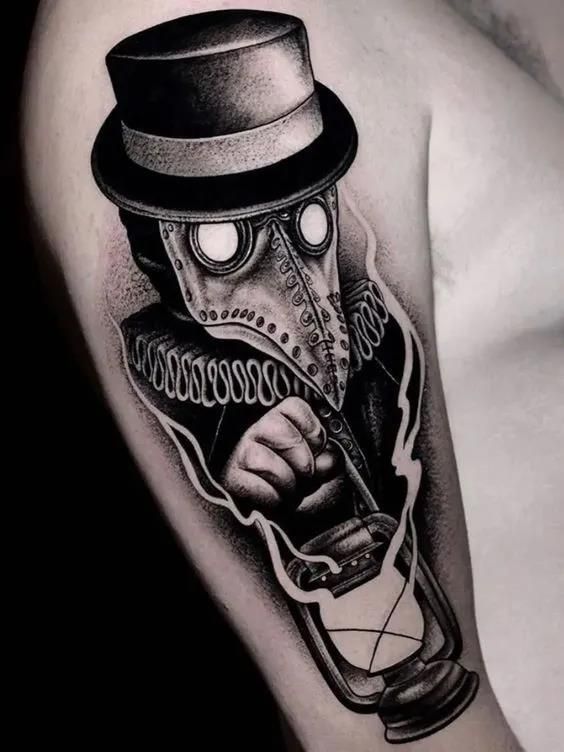The vertically aligned, black-and-white photograph exhibits a man's right bicep adorned with an intricate tattoo. Dominating the left side of the image is a solid black space, contrasting starkly with the detailed art on the man's arm. The tattoo extends from his shoulder down to his elbow, where the image cuts off. The central figure of the tattoo is a humanoid creature with distinctive avian features, including a pronounced beak and empty, white eyes framed by small black goggles. Atop its head rests a black top hat with a ribbon, and it is clad in a black jacket, possibly with a clown collar. In its right hand, the figure holds an old-fashioned lantern, which dangles down to the elbow, rendered in black and grayish shades. A glimpse of the man's chest hair is visible in the upper right corner of the picture, further grounding the focus on the tattooed arm.